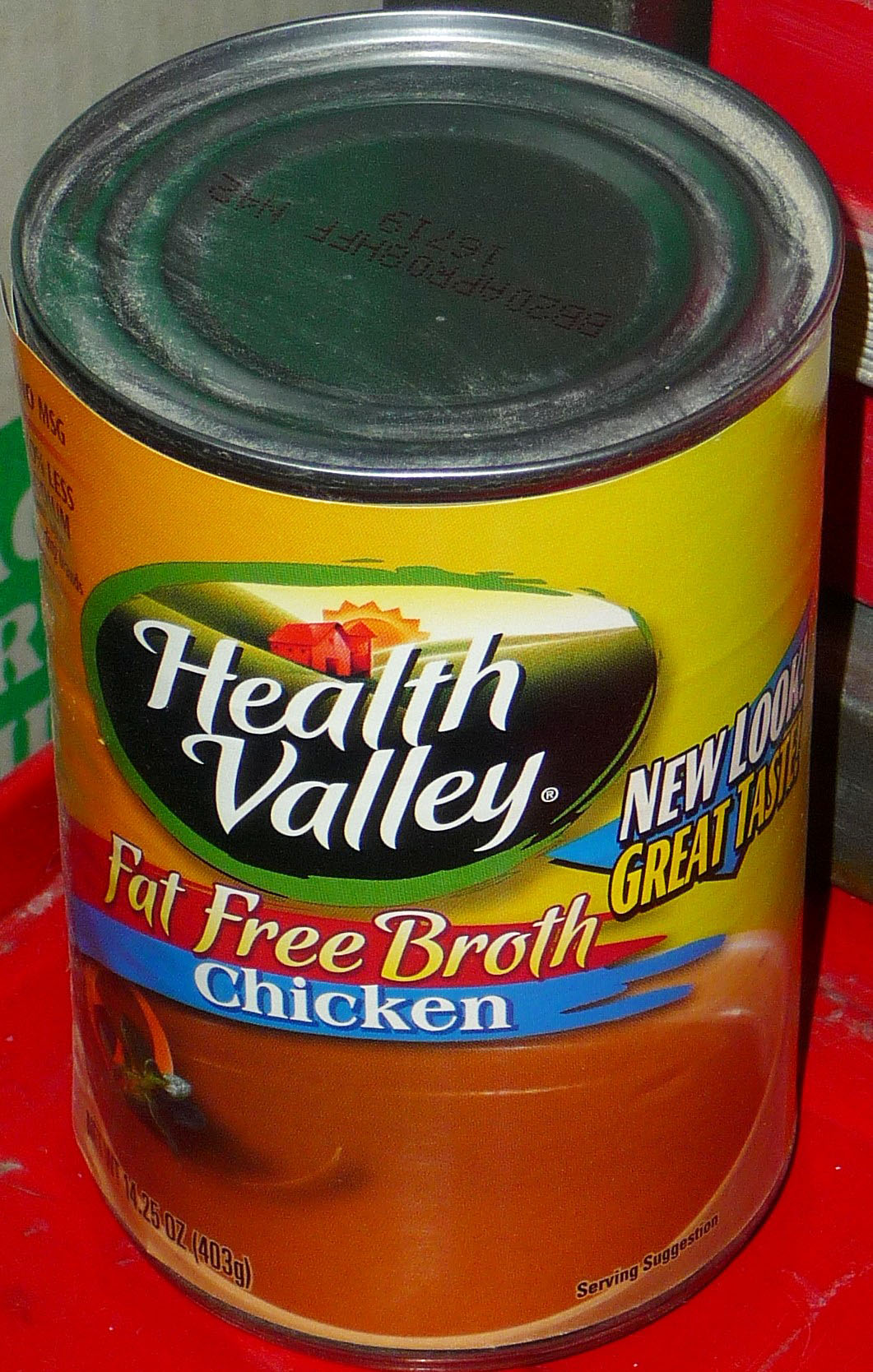A close-up image features a can of Health Valley Fat-Free Chicken Broth placed on a red plastic tray. The can, showcasing a new look and promising great taste, is notably dirty on top, suggesting it has been stored in a dusty area. This indicates the necessity of checking the expiration date before use. The overall color scheme of the can is predominantly yellow. The Health Valley logo, situated near the top, is framed within a roughly oval green shape, depicting a sunrise over a verdant valley. The broth inside the can appears more red than clear, possibly influenced by the vibrant red tray, giving it an unappetizing appearance that might deter trust in the brand.